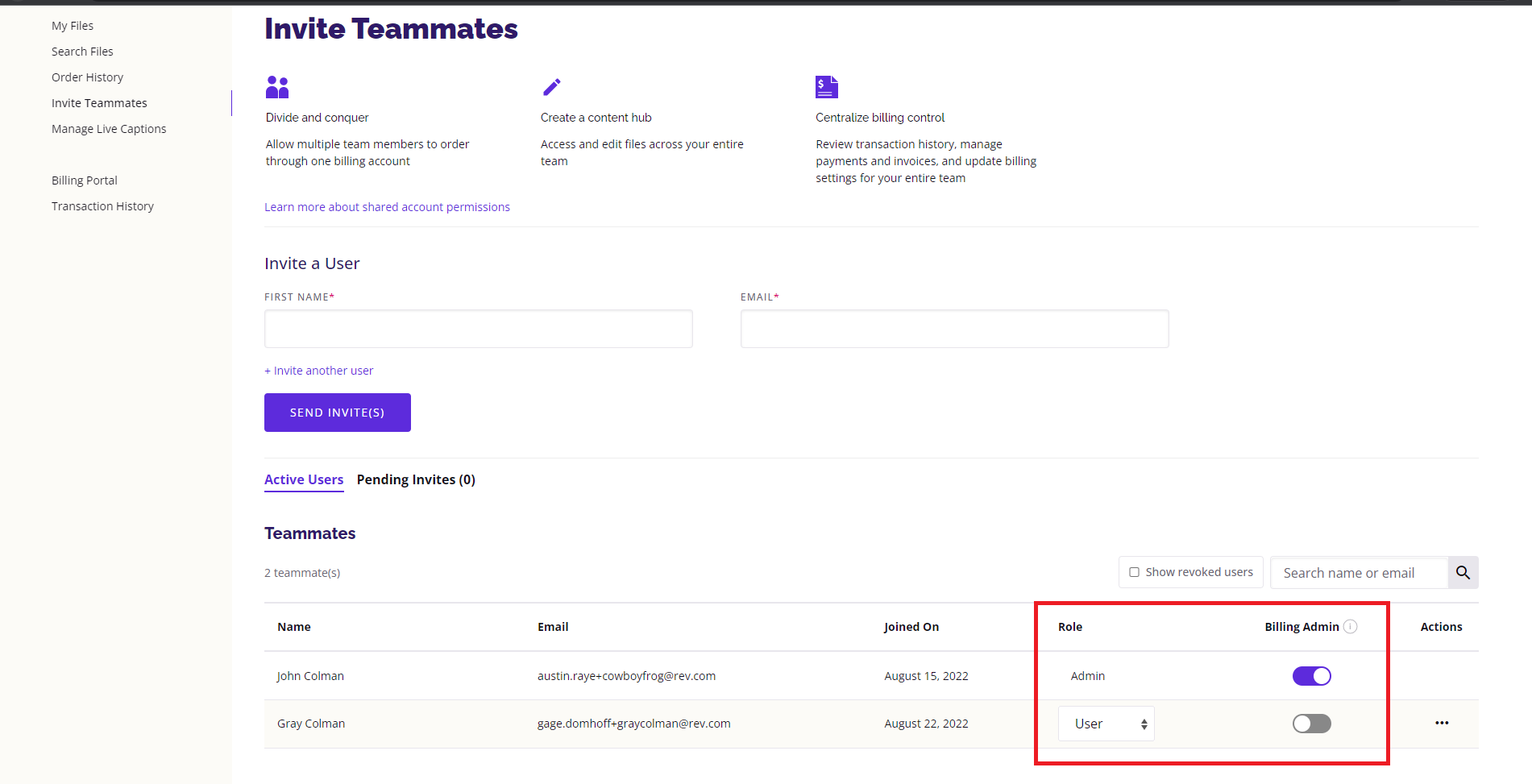This is a detailed screenshot of a team management interface. At the top, in bold black text, it says "Invite Teammates." On the left margin, several navigation categories are listed:

- **My Files**
- **Search Files**
- **Order History**
- **Invite Teammates** (currently selected)
- **Manage Live Captions**
- **Billing Portal**
- **Transaction History**

Below "Invite Teammates," three main categories are listed with their respective purple icons:

1. **Divide and Conquer**
2. **Create a Content Hub**
3. **Centralize Billing Control**

Each category is explained in detail:
- **Divide and Conquer:** Allow multiple team members to order through one billing account.
- **Create a Content Hub:** Access and edit files across your entire team.
- **Centralize Billing Control:** Review transaction history, manage payments and invoices, and update billing settings for your entire team.

Below the explanations, there is an option to invite a user, with two input fields—one for the first name and another for the email address. Beneath these fields, in purple text, it says "Invite Another User," followed by a purple box with white text that reads "Send Invites."

Towards the bottom of the screenshot, there are sections for "Active Users" and "Pending Invites," both currently showing zero. "Active Users" is highlighted in purple. Within this section, it lists:

- **Teammates**: Shows two teammates.
- Options to "Show Revoked Users" and a search field labeled "Search Name or Email."

Underneath these options, there are three categories in black text: Name, Email, and Joined On. Two names are listed under these categories.

On the right side of the list, the "Role" category is highlighted with a red rectangular border. Within this category, there are two options: "Admin" and "User." The "Admin" button has been toggled on, indicated by a purple button with a white circle on the right, while the "User" button remains unselected.